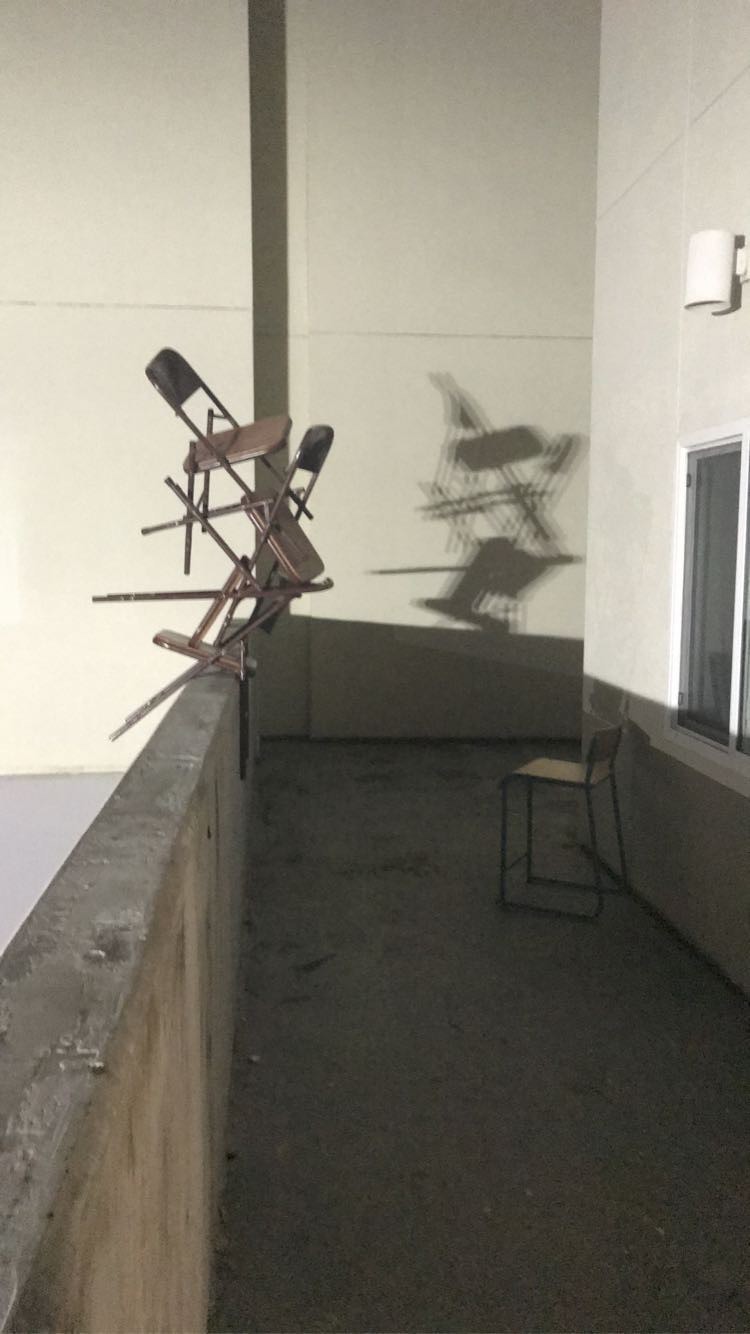In this black and white image, we see an exterior scene that appears to be taken from a balcony or ledge of a building. The beige walls in the background are accented with a white-framed window, above which there is a small light fixture. The image is characterized by intentional art-like quality emphasizing contrast and shadows. 

On the dark cement floor, which casts its own shadow, we find a distinctive brown chair with black legs positioned to the right. Central to the scene, however, is a stack of three metal folding chairs, which despite their precarious placement, are meticulously balanced on the waist-high cement railing to the left. These chairs, described as rusted and steel, create a striking composition as light from the left illuminates them, casting intricate, intertwined shadows on the wall behind. 

The overall setting suggests a thoughtfully composed artistic photograph, showcasing the interplay of light, shadow, and texture in a seemingly ordinary scene transformed into an abstract visual narrative.